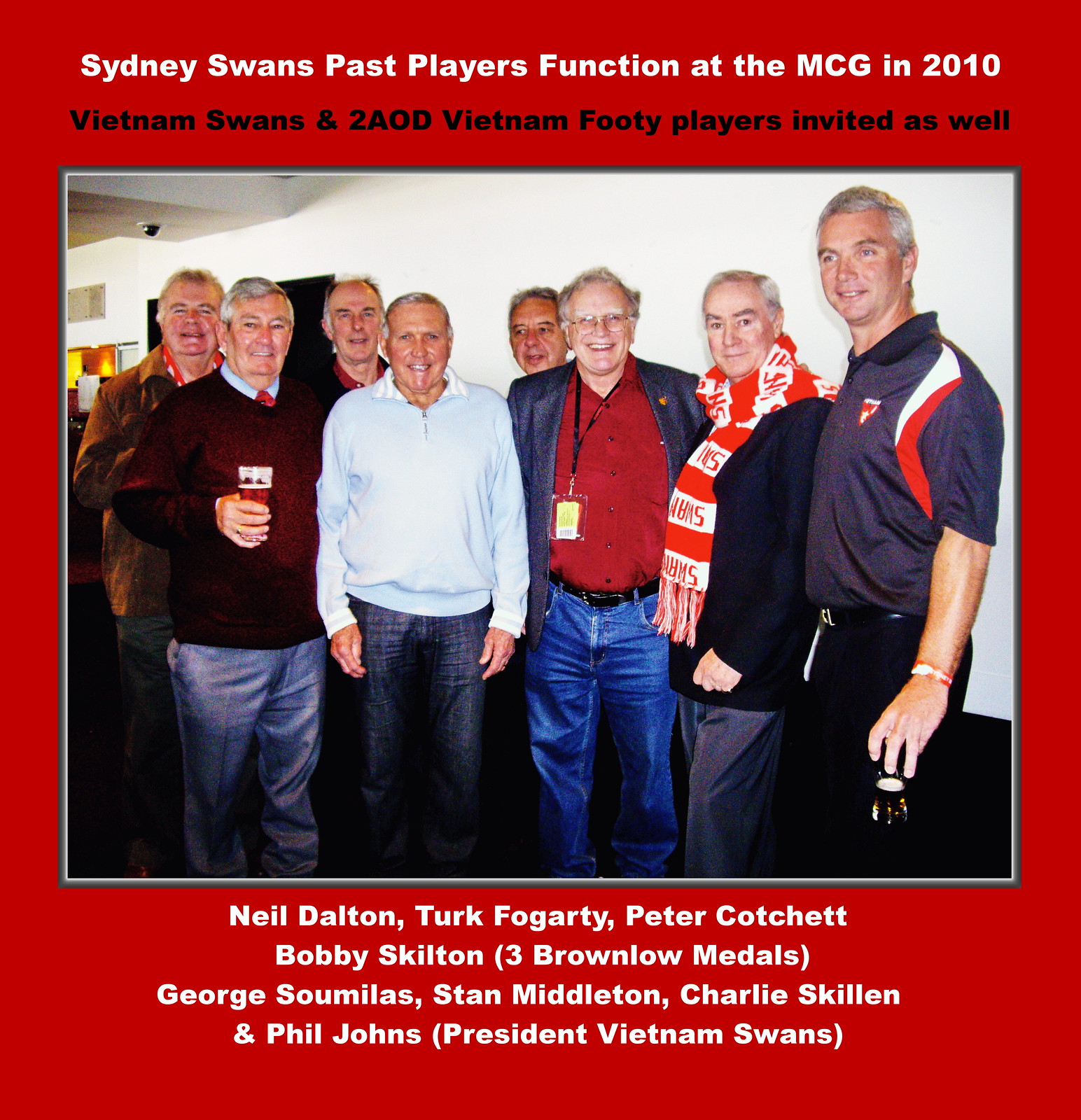A vibrant color photo captures a reunion of former Sydney Swans soccer players, taken at the MCG in 2010. The image is centrally framed by a red border. At the top, white text reads, "Sydney Swans Past Players Function at the MCG in 2010," followed by black text stating, "Vietnam Swans and two AOD Vietnam footy players invited as well." The group of about ten older gentlemen, mostly sporting gray hair, stand shoulder to shoulder, all smiling for the camera. They are dressed casually, with a mix of sweaters and jeans, underscoring the possible winter setting. One man on the left side holds a pint of beer in his right hand, and another features prominently with a red and white scarf. Behind them, there's a white wall, making the gathering appear as if it could be in a brewery or similar venue. Below the photo, white text lists the names and titles of these distinguished individuals: Neil Dalton, Turk Fogarty, Peter Kochet, Bobby Skilton (three-time Brownlow Medallist), George Samolis, Stan Middleton, Charlie Skillen, and Phil Johns (President, Vietnam Swans).